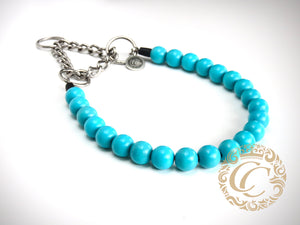The image features a stunning bracelet adorned with solid, light blue circular beads that exude a distinctive shade reminiscent of Aztec or Incan art. These opaque beads are meticulously arranged and connected by a silver metallic chain forming a triangular shape at the top left corner, complete with shiny silver clasps. The bracelet is elegantly laid out on a white surface that subtly transitions to a darker gray at the corners, emphasizing the bracelet as the focal point. Dominating the bottom right corner of the image is a gold ornate logo, displaying two stacked "C's" encircled by a vine floral border, adding an intricate touch to the overall simplicity and beauty of the design.